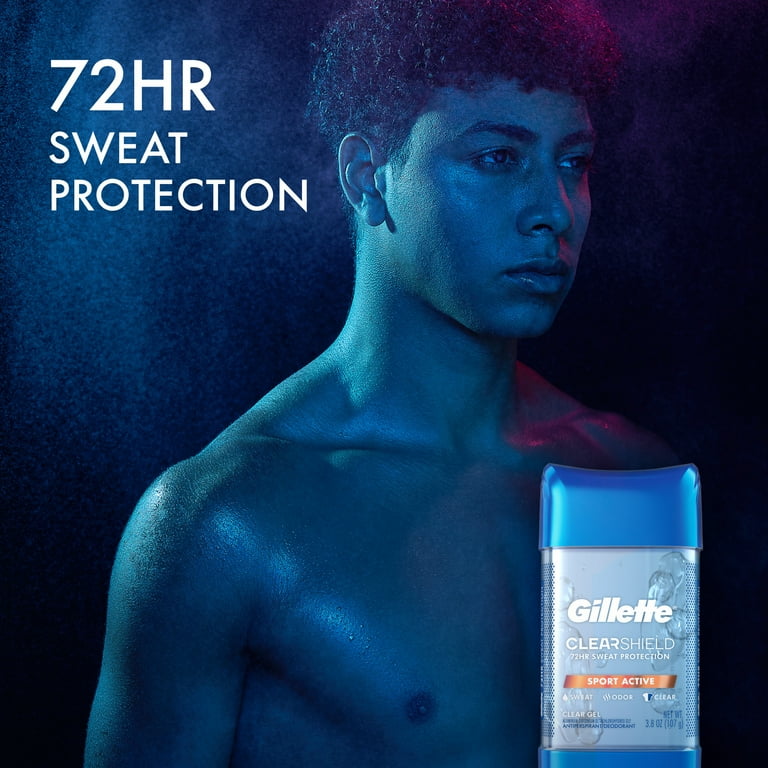The advertisement is for Gillette Clear Shield Antiperspirant Gel, specifically designed for sport-active men, offering 72-hour sweat protection. The product is displayed in the bottom right corner, in a clear bottle with a black cap and a blue base, and it weighs 3.8 ounces (107 grams). The background features a young, shirtless African-American man with a glistening, muscular physique, suggesting he is sweating. He has curly, short afro hair and gazes to the right of the image. In the upper left corner, white text prominently states “72 hours sweat protection” against a backdrop of blue, black, and purple hues, emphasizing the product's long-lasting effectiveness in combating sweat and odor during intense physical activity.